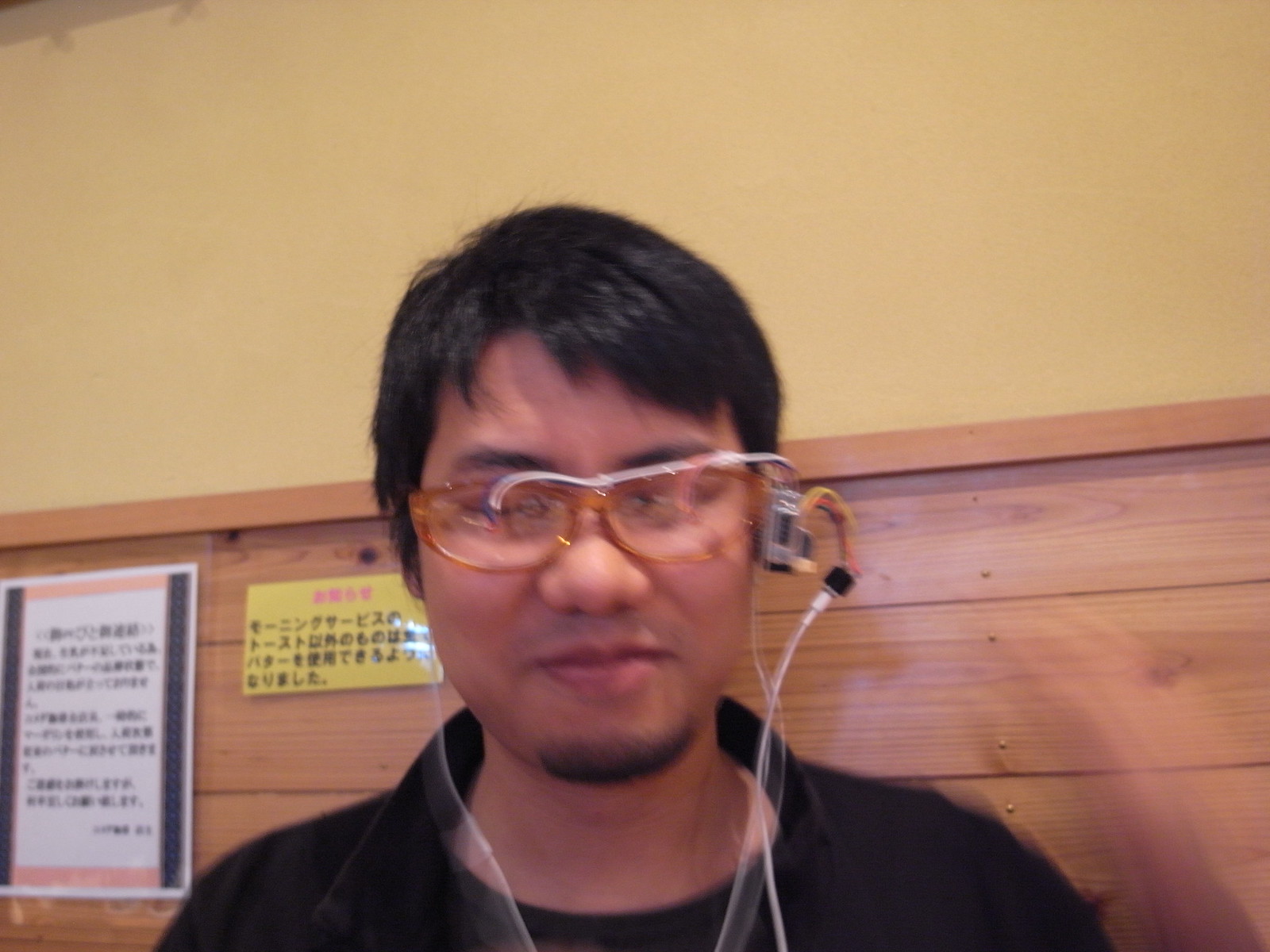The image features an Asian man with short dark hair, dark eyebrows, a short goatee, and a wide nose. He wears eyeglasses with an unusual apparatus attached to them. This apparatus includes a small silver box near his ear and a curved, upside-down U-shaped orange component. The orange arm has a small black fixture at its end, with a cable extending downward off the bottom of the screen. Additionally, there is a white tube running across the top of his glasses, and he has earbud-like earphones connected to a white cord. The man is dressed in a black, collared shirt and a black jacket.

He stands in front of a wooden wall, constructed of brown planks with visible grains, knots, and even some screws. This wall extends to about the middle of his head, suggesting it is approximately five and a half feet tall. Above the wooden section, the wall is yellow.

On the wooden wall, there are two signs. One is a white piece of paper, approximately 8x11 inches, featuring an orange border at the top and bottom, black stripes along the sides, and filled with Chinese writing. The other sign is a larger yellow rectangle with a single line of red writing at the top and four lines of black writing below, all in Chinese.